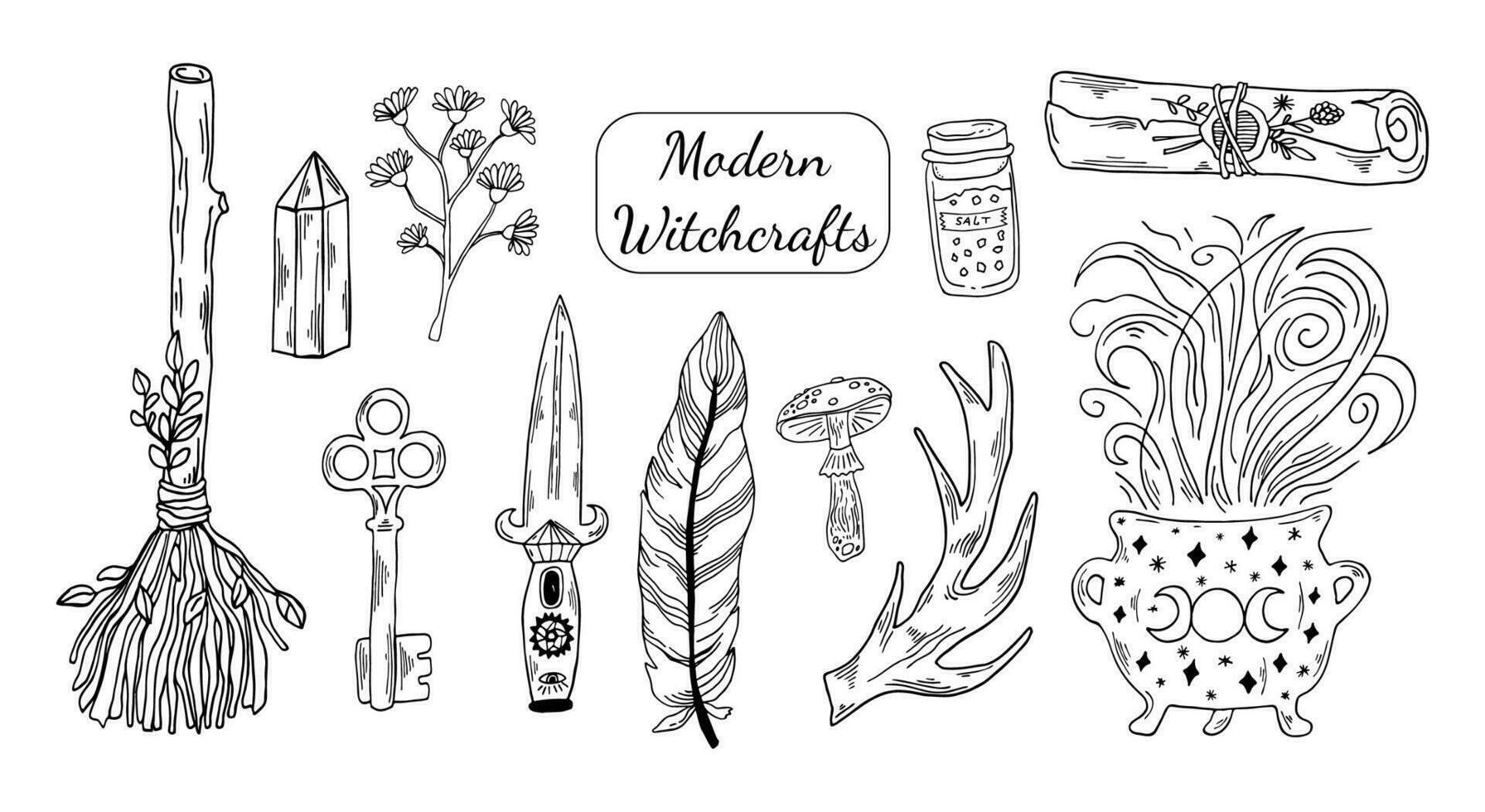This black and white illustration features a central rectangle framed in a decorative border, containing the cursive text "Modern Witchcrafts." Surrounding this text are meticulously drawn witchcraft-related items. On the left, a broom crafted from a branch is visibly tied with leaves at the base. Adjacent to the broom, a detailed crystal is depicted. Beneath the crystal is an old-fashioned key with three round holes at the top. Nearby, a delicate twig with flowers on the ends is shown, followed by an intricately designed dagger featuring the all-seeing eye on its handle. Further right, a large feather, a mushroom, and a bottle of salt resembling an antler or horn are displayed. Finally, there's a cauldron with swirling steam and flames beneath it, and it is decorated with a moon, a sun, and another moon design. All the objects are rendered with minimal shading on a stark white background, highlighting their distinct and detailed characteristics.